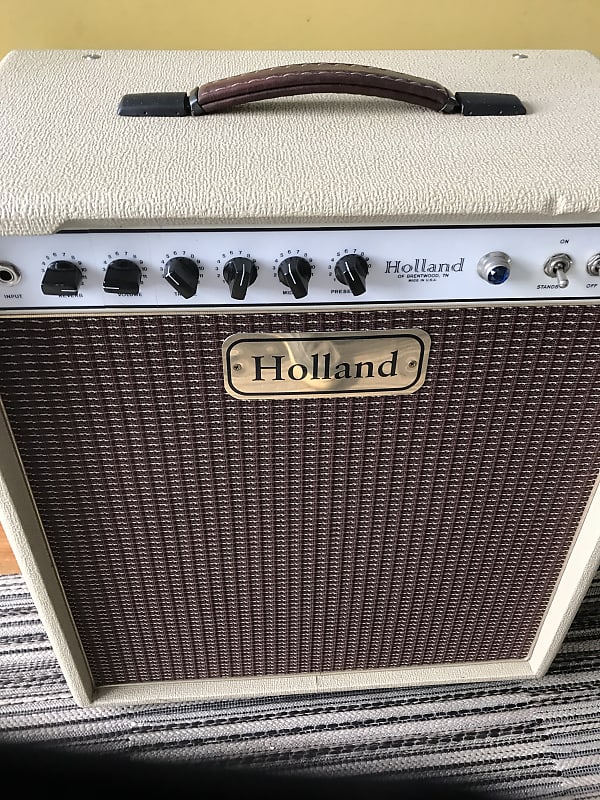This is a somewhat top-down photograph of a vintage Holland music amplifier, likely used for electric guitars, basses, or other electric instruments. The amplifier is sitting on a black and white rug, with a yellow strip of wall visible at the top of the image. The amplifier itself features a distinctive design with an off-white top and a brown leather handle. The front of the amp displays a brown grill with a gold and black metallic nameplate that says "Holland." 

The control panel located on the top section of the amplifier is white and houses several black knobs labeled with black numbers, presumably for adjustments such as volume, gain, and reverb. There is also a silver input jack on the far left, a black standby toggle switch, and an on/off switch towards the right. The white surface of the amp has a rough texture, adding to its vintage appeal. Despite a small dent in the upper right-hand portion, the amplifier appears to be in excellent condition, suggesting it has been either well-maintained or refurbished. The amp also features additional branding details such as "Holland of Brentwood, Tennessee, made in USA" near the right side of the control panel.